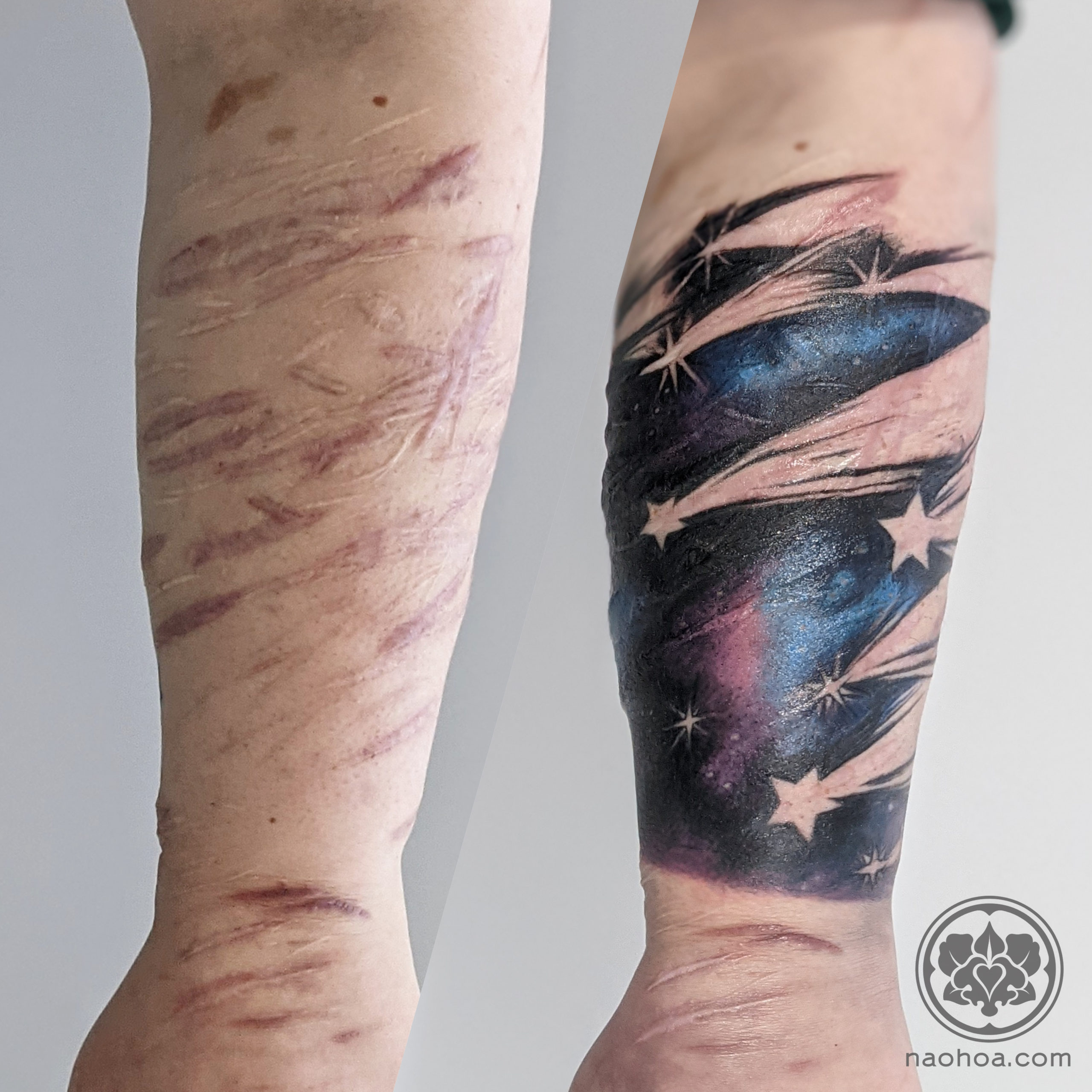The image displays a detailed before-and-after comparison of a person's forearm that has undergone a significant transformation. The left side of the photo reveals the forearm marred with red scars, indicative of previous self-harm. In stark contrast, the right side showcases a beautifully crafted tattoo that expertly covers these scars. The tattoo features a celestial nighttime scene, rich with dark blue and black hues resembling a starry sky. Interspersed throughout are stars created using negative space, about six in total, giving the effect of shooting stars across the forearm. Every intricacy of the celestial design—from the metallic hints of nighttime blues to the skin-colored stars—helps to mask the underlying blemishes effectively. In the bottom right corner of the image, the logo "naoha.com" appears, depicting a heart intertwined with a plant.